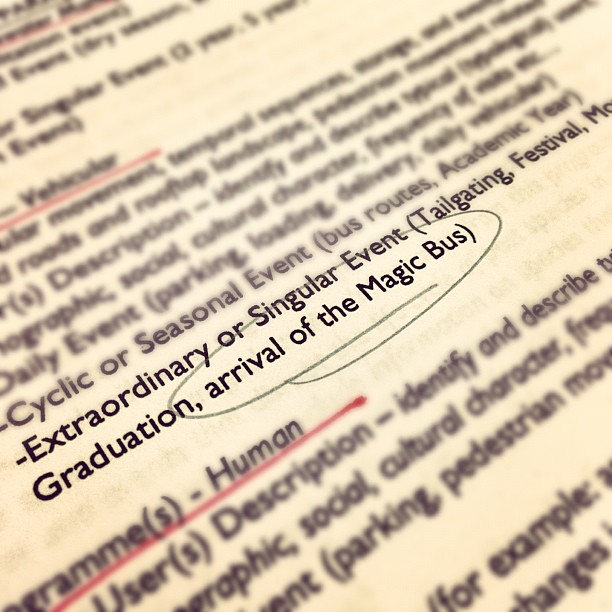This image displays a close-up shot of black text on white paper, resembling a page from a book, magazine, newspaper, or article. The text is angled, slanting from the top left to the bottom right. Most of the text is blurred, making it difficult to read, except for two lines that are clearly visible and appear to be the focal point of the image. These lines read "Extraordinary or Singular Event" and "Tailgating Festival," with the most significant phrase being "Graduation, Arrival of the Magic Bus," which is circled in black ink. This circled text is centrally positioned and highlighted as the primary focus of the image, emphasizing its importance in the context. The color scheme includes shades of black, white, and off-white, giving the impression of traditional print media.